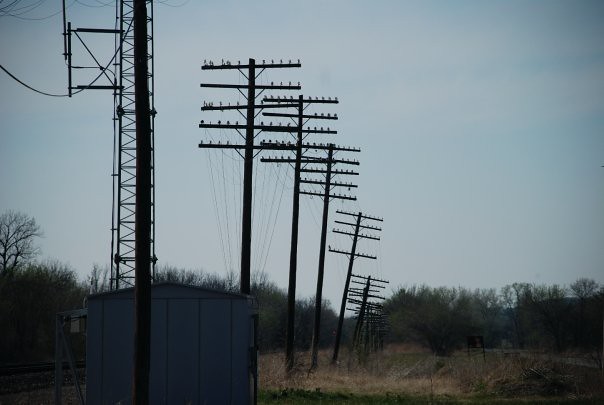This photograph captures a row of tall, slender utility poles, extending into the distance across a dry, grassy field. The poles, which feature five horizontal bars at the top, appear to diminish in size as they recede into the distance, giving the impression of a slight lean to the right. These black cylindrical poles are strung together by thin power lines, forming a line that is positioned prominently on the left-hand side of the image. In the foreground, there's a small, bluish-gray metal shed located at the bottom left corner. The scene is set under a blue sky dotted with white clouds, and the landscape is framed by trees with no leaves, creating a sense of an unkempt, yet serene environment.